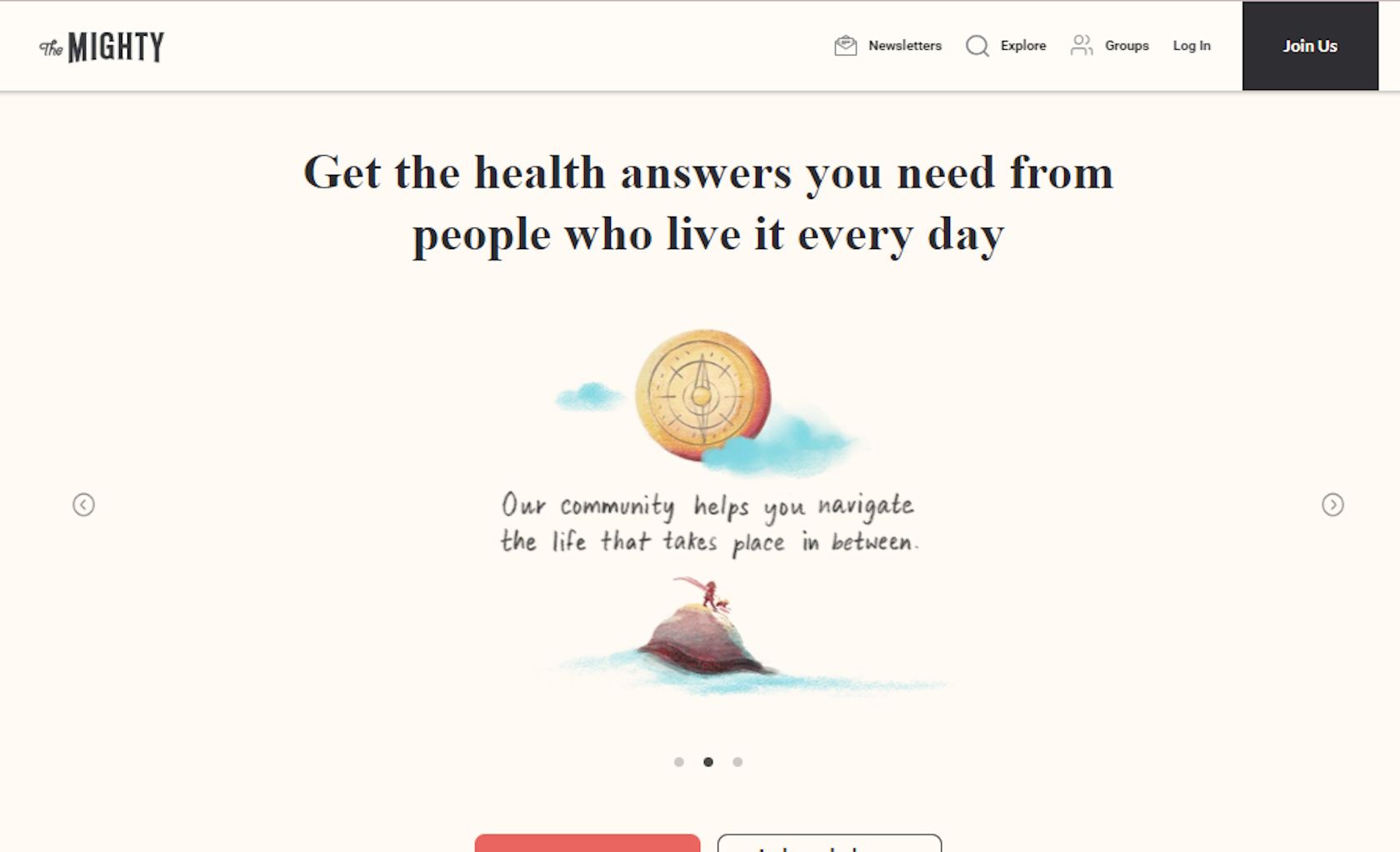The top of the webpage features a header with the title "The Mighty" prominently displayed in the upper-left corner. On the far right side of the header, there is a row of icons and links, including an envelope icon labeled "Newsletters", a magnifying glass icon labeled "Explore", an icon with people labeled "Groups", and a simple text link that reads "Log In". Further to the right, in a black box with bold white text, there is a call-to-action that says "Join Us".

Moving down to the center of the page, the main message reads: "Get the health answers you need from people who live it every day". Below this, there is an image of a compass amidst clouds, accompanied by the text: "Our community helps you navigate the life that takes place in between". Further down, there is a watercolor painting of a rock with two tiny figures standing on it. On either side of this central image, there are left and right carets (arrows) that allow users to cycle through different pictures.

At the bottom of the visible screen, there are two buttons, but only the top halves of these buttons are visible, indicating that additional content can be found by scrolling further down.